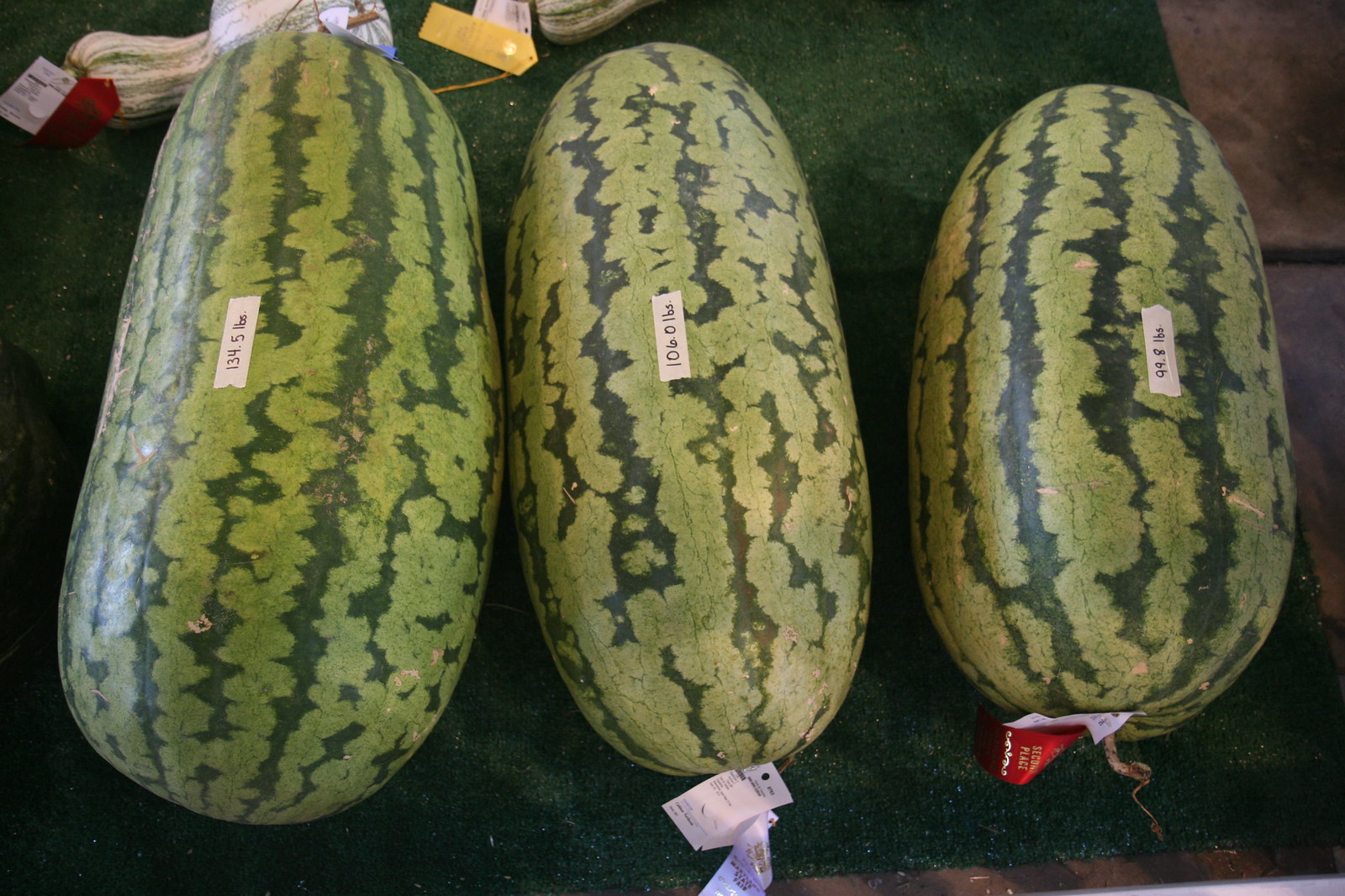The image features three giant watermelons placed side-by-side on a dark green tarp-like fabric. Each watermelon bears a small white label in the very center, listing their weight: the leftmost watermelon is labeled as 134.5 pounds, the middle one as 106.0 pounds, and the rightmost one as 99.8 pounds. These labels are written in black marker on the white tape. The melons are of a light green color adorned with dark green, almost black, stripes running vertically. The setting suggests a contest with the watermelons possibly winning different awards; a red ribbon is attached to the rightmost watermelon and a white ribbon to the middle one. A small portion of gray flooring is visible on the right side of the image, and a series of cut-off small objects, including a visible yellow tag, appear at the top. The watermelons are extremely zoomed in, taking up most of the picture and prominently displaying their textures and weights.